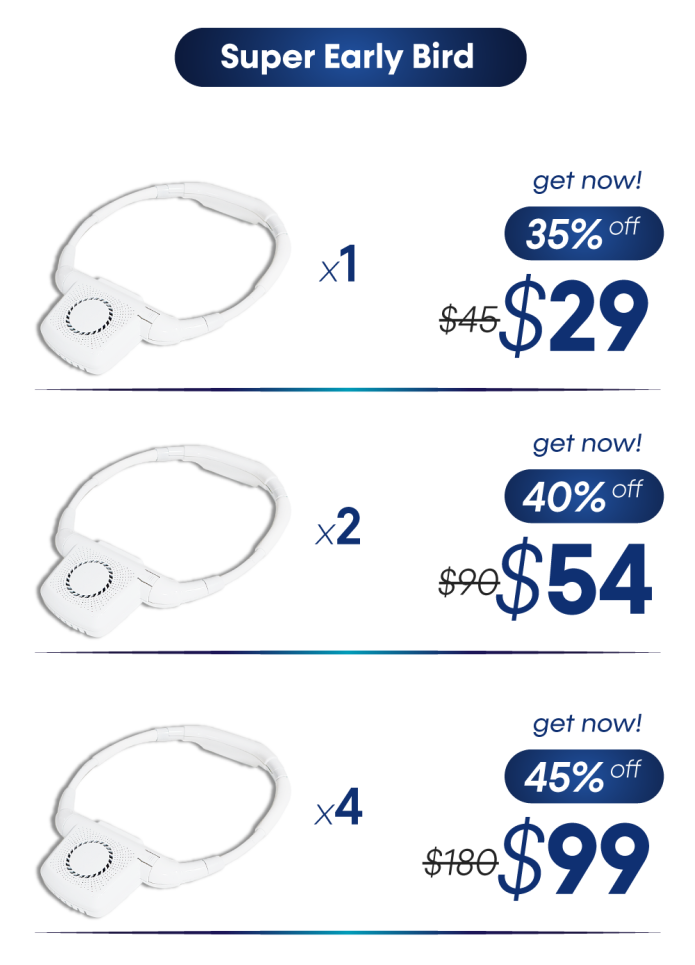At the top of the image, there is an illustration of a bee. Below the bee, there is a blue oval with the text "Super Early Bird" inside it. To the right of the blue oval, there is an icon that could either be a lock or a faceplate. Underneath this icon, there is a square section featuring what appears to be a white plastic device with fan-like features. 

To the right of this device, there is text that reads "X1" indicating a quantity of one. Below this, there is a button labeled "Get Now," alongside a discount offer "35% off," with the original price "$45" slashed through and a discounted price of "$29" prominently displayed.

Next, there is an item that appears to be a plastic device labeled "X2," indicating a quantity of two. This is followed by the text "$90," a dash mark, and another "Get Now" button. The offer next to it states "40% off," with the original price scratched out and marked as "$54" in blue text. 

Another dividing line in blue follows this section, leading to a description of another plastic device labeled "X4," indicating a quantity of four. This is accompanied by a "Get Now" button with a discount label "44% off." The original price "$180" is scratched out and replaced with the discounted price of "$99."

Overall, the image conveys that the more units you purchase, the greater the discount you receive.